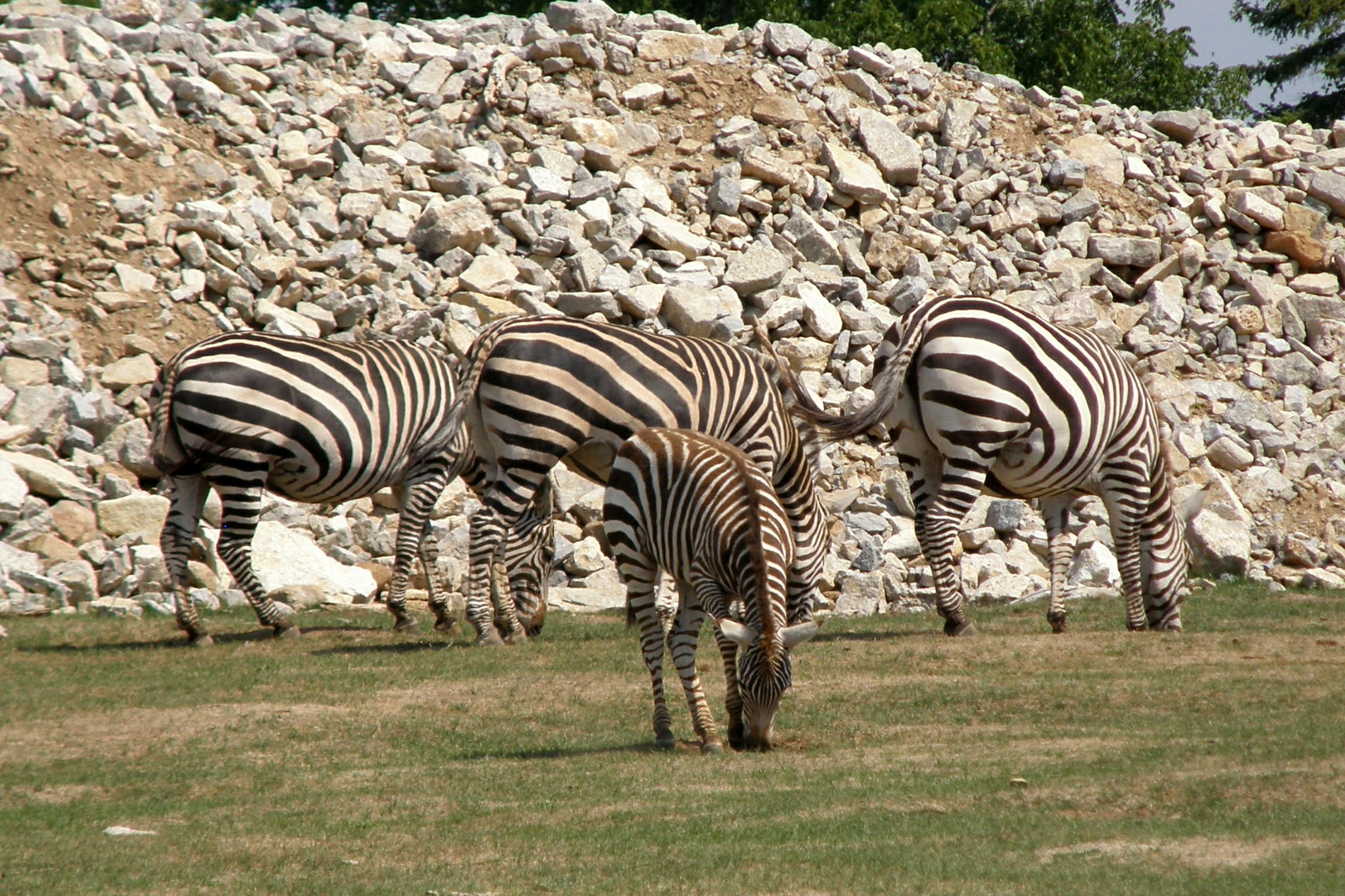This detailed image captures a small herd of four zebras grazing on a grassy field that has a mix of green and patches of brown grass. The scene is set toward the base of a large, rocky hill that is covered mostly with big, gray boulders and some brown dirt. These rocks appear precariously close to the leftmost zebra, suggesting they could easily slide down and pose a danger. Three of the zebras are adults, characterized by their robust, black and white striped bodies, with some having a brownish tinge to their stripes. Their tails appear braided, blending black and white stripes before ending in straight hairs. All three adult zebras face away from the camera with their heads down in the grass. The fourth zebra, smaller and likely an adolescent, is positioned in front of the adults. It has a more brownish and white coloration, and also has its head down grazing. The terrain extends upward from the zebras to the rocky hill, and the backdrop features a glimpse of green leafy trees and a patch of blue sky, which hints at a wider landscape beyond.